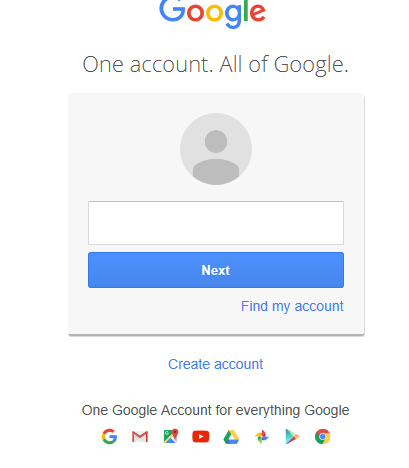This image features the main page of Google, showcasing its widely recognized logo with the letters in vibrant blue, red, yellow, green, and orange colors, reflecting Google's typical branding. At the center of the page, the familiar tagline "One account. All of Google." emphasizes the integration of services. Below this, there is a prominent empty search field. 

To the right of the search field, buttons labeled "Find my account" and "Create account" are visible, highlighting the ease of accessing or initiating a Google account. The footer of the page displays various colorful app icons representing multiple Google services, including Google Search, Gmail, Google Maps, YouTube, Google Drive, Google Photos, the Google Play Store, and Google Chrome, reinforcing the "one account for everything" concept. The background of the page is a clean, crisp white, ensuring that all elements stand out clearly.